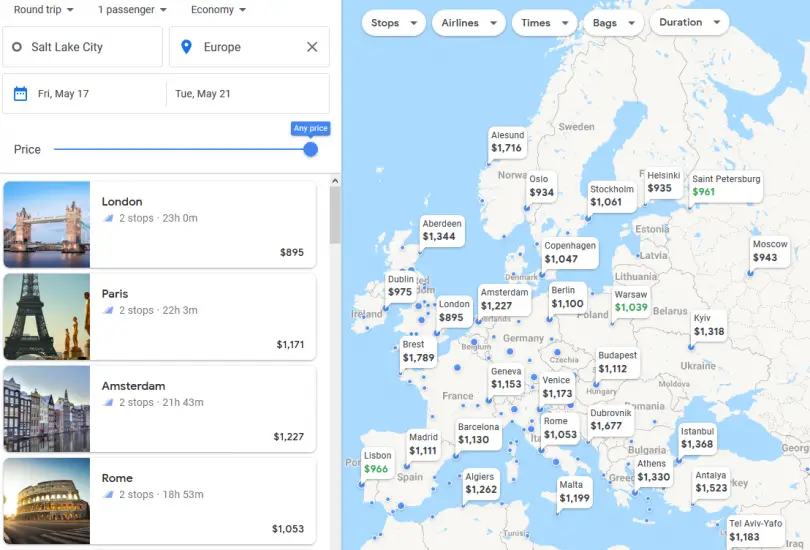Photographic image taken from a web page showcasing a flight search interface for a round-trip, one passenger, economy class journey.

On the left side of the interface, several drop-down menus are visible. One menu shows the departure city as Salt Lake City and the destination as Europe. The travel dates are Friday, May 17th through Tuesday, May 21st. Below the drop-down menus, a price slider is clearly marked, with the selected option set to ‘Any Price’ in blue.

Detailed search results for various European destinations are displayed:
- **London:** The image includes the iconic Tower Bridge. The flight involves two stops, with a total duration of 23 hours and 0 minutes, costing $895.
- **Paris:** The Eiffel Tower is featured in the image. This option also has two stops, with a total travel time of 22 hours and 30 minutes, priced at $1,171.
- **Amsterdam:** An image of the city buildings alongside a waterway is shown. This route requires two stops, with a total duration of 21 hours and 43 minutes, costing $1,227.
- **Rome:** The Colosseum is depicted. This flight involves two stops, taking a total of 18 hours and 53 minutes, with a ticket price of $1,053.

To the right of the search results, there is a map of Europe, visually representing the destinations.